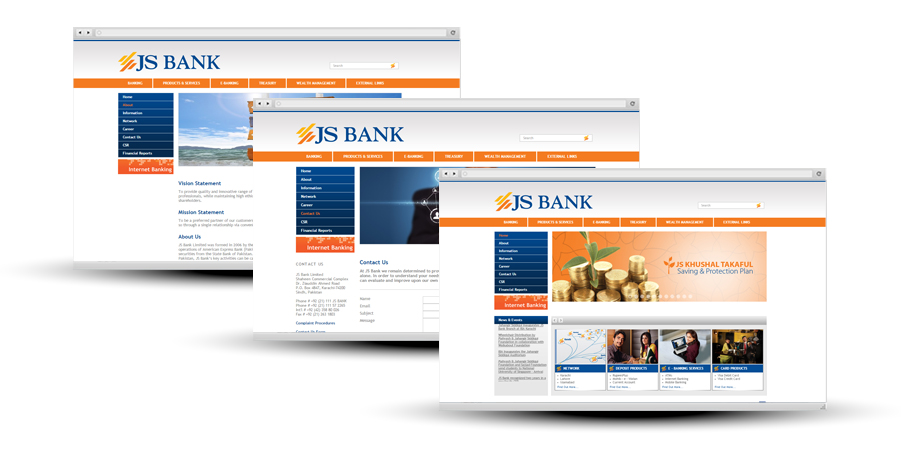The image showcases a computer screen displaying three overlapping webpages from JS Bank, fanned out diagonally from the upper left to the lower right. The front page, prominently placed in the lower right corner, is fully visible, whereas the other two pages are partially obscured, with only portions revealed.

Each webpage features "JS Bank" in bold blue font, accompanied by orange and yellowish-orange decorative lines, possibly part of the emblem. At the top of each page, a horizontal orange bar contains clickable areas. The left sidebar on all pages includes interactive sections within blue rectangles with white text and additional sections within orange rectangles.

On the webpage positioned at the back, there are visible sections labeled "Vision Statement," "Mission Statement," and "About Us." The middle webpage reveals a "Contact Us" section. The frontmost webpage prominently displays the text "JS Kuchel," likely referring to a specific service or plan, described as a "savings and protection plan."